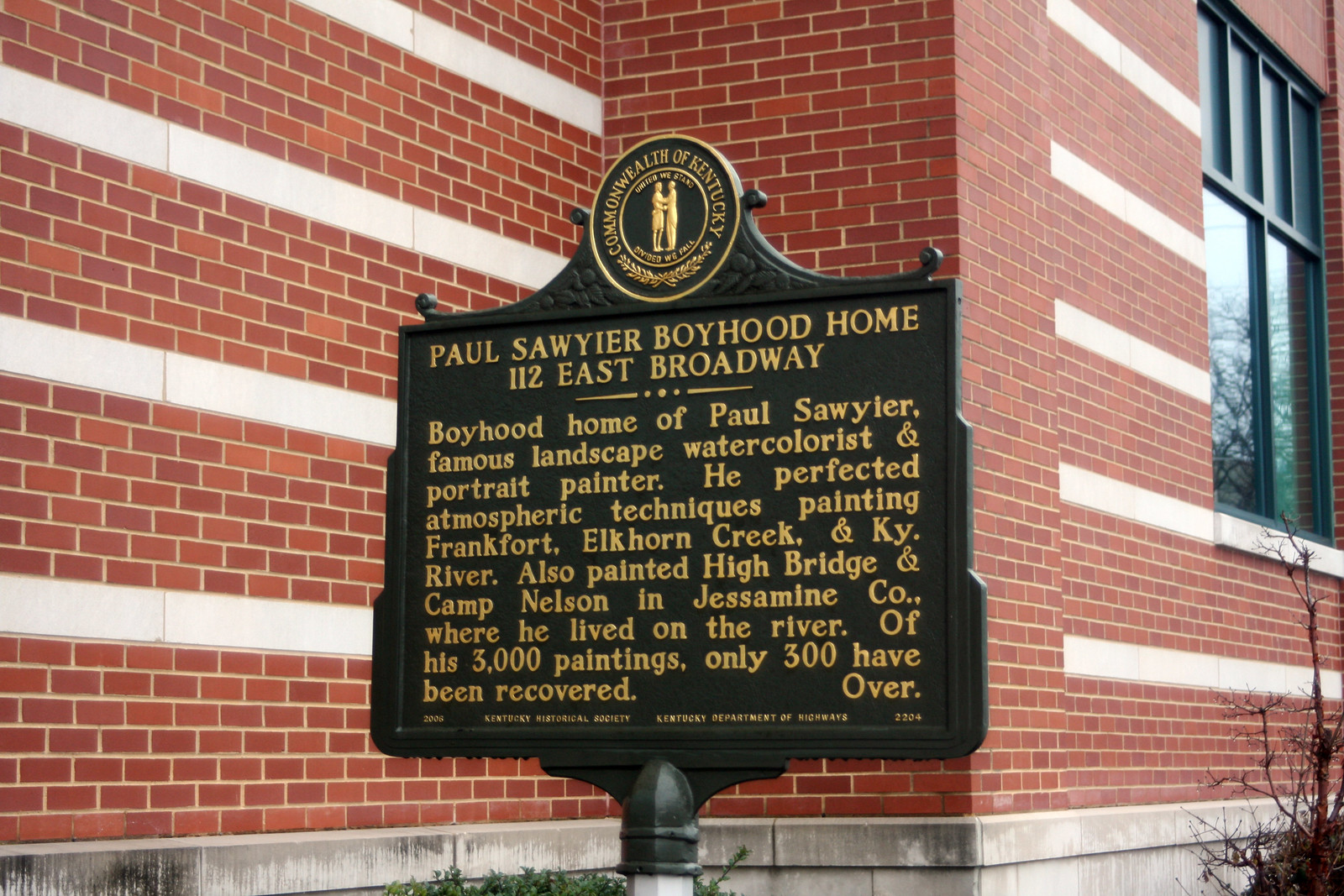The image features a historical red brick building with dark metal-framed windows and lighter-colored horizontal brick stripes. In front of the building stands a black metallic plaque with gold lettering, mounted on a post. At the top of the plaque is an embossed logo of two people embracing, encircled by the words "Commonwealth of Kentucky" and "Divided we fall." The plaque reads: "Paul Sawyier Boyhood Home, 112 East Broadway. Boyhood home of Paul Sawyier, famous landscape watercolorist and portrait painter. He perfected atmospheric techniques painting Frankfort, Elkhorn Creek, and Kentucky River. He also painted High Bridge and Camp Nelson in Jessamine County, where he lived on the river. Of his 3,000 paintings, only 300 have been recovered." At the bottom of the plaque, it reads: "Kentucky Department of Highways, Kentucky Historical Society," with the word "Over" indicating more information on the reverse side.